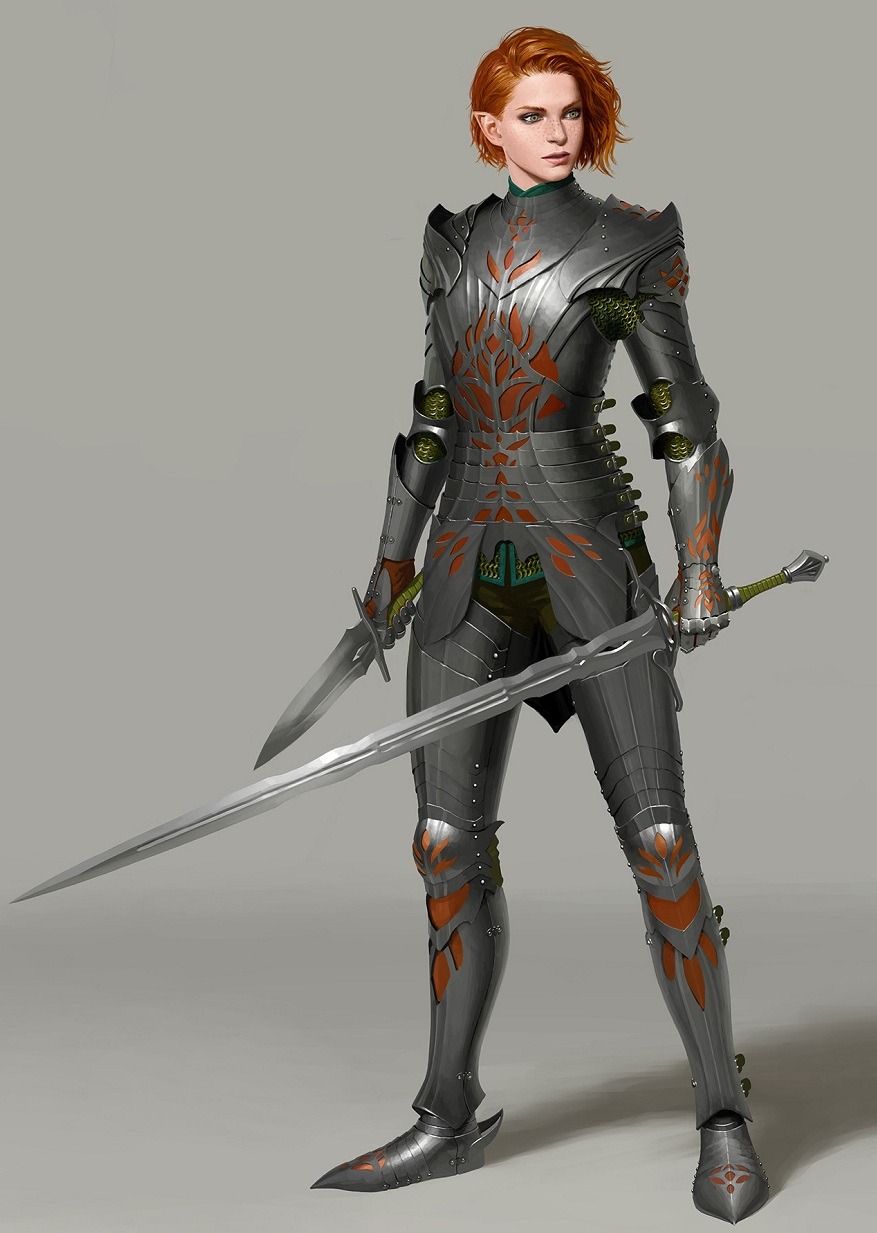This is a highly detailed digital illustration of a fierce fantasy female warrior with an elven appearance, signified by her pointed ear visible beneath her short, ginger-red hair that swoops back from her face. She has a fair complexion adorned with freckles, expressive grayish green eyes, and pink lips. Her meticulously designed armor is primarily grayish silver, decorated with intricate patterns resembling orange petals and leaves. There are also notable splotches of black and an almost stained glass-like effect of bronze or brown throughout the armor. Beneath the plated armor, gaps reveal brass-colored chainmail accented with green, further protecting her arms and shoulders. She dons gray metal plated leggings and boots, each embellished with the same orange decorations seen on her armor. 

In her left hand, she wields a large silver broadsword, and in her right, she holds a matching silver knife, both with handles wrapped in green twine. A dark green tunic with light green accents can be seen under her armor, adding layers to her formidable ensemble. The entire scene is set against a simple gray background, with shadows cast at her feet, enhancing the realism of this enchanting character.